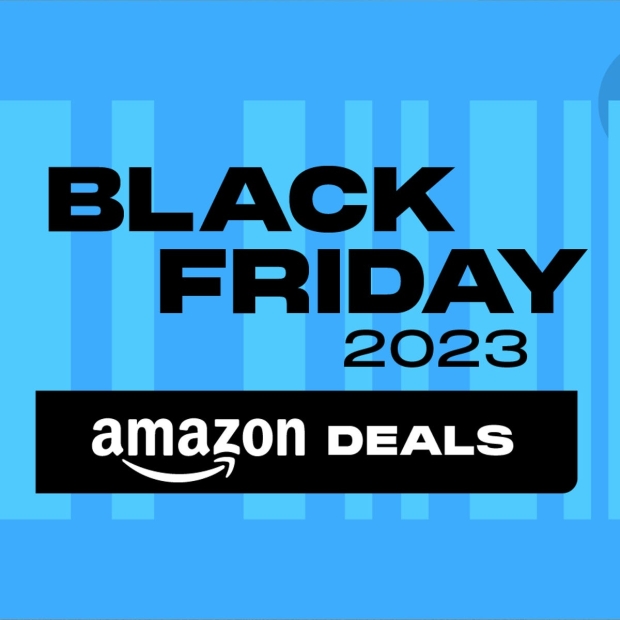The image appears to be a screenshot of an online pop-up advertisement for Amazon's Black Friday 2023 deals. The background is a large, light blue square filled with vertical lines in varied shades of blue, creating a barcode-like effect. These vertical lines differ in width, alternating between thick, thin, and medium, enhancing the overall textured appearance. 

Centrally placed on this backdrop are the words "Black Friday 2023," formatted in a stylish manner with "Black" left-aligned, "Friday" right-aligned on the subsequent line, and "2023" positioned a space or two in from the right edge. Directly below this text is a black, rectangular banner with the iconic white Amazon logo, featuring the characteristic arrow stretching from 'A' to 'Z', followed by the word "deals". The design and layout suggest this pop-up ad aims to attract attention to Amazon's specials for Black Friday.